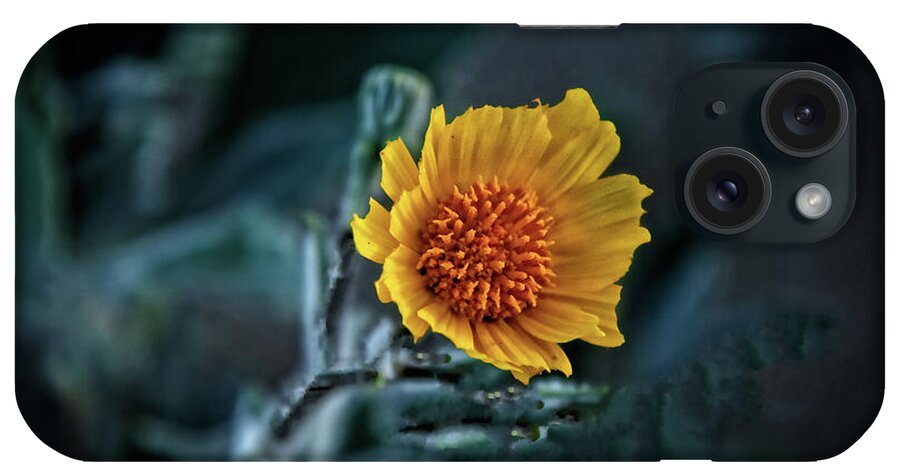The image depicts the back of a newer model smartphone, likely an iPhone, placed horizontally. Dominating the center of the phone case is a bright yellow flower, possibly a daffodil or dandelion. The flower features vibrant yellow petals with intricate orange sepals at its core. The background of the phone case consists of a mix of dark greens, blues, and aquas, giving a somewhat abstract and dark appearance. In the upper right-hand corner, the dual camera lenses and flash of the phone are visible, suggesting it's a modern iPhone. The design does not include any text, focusing instead on the detailed and vivid floral centerpiece.